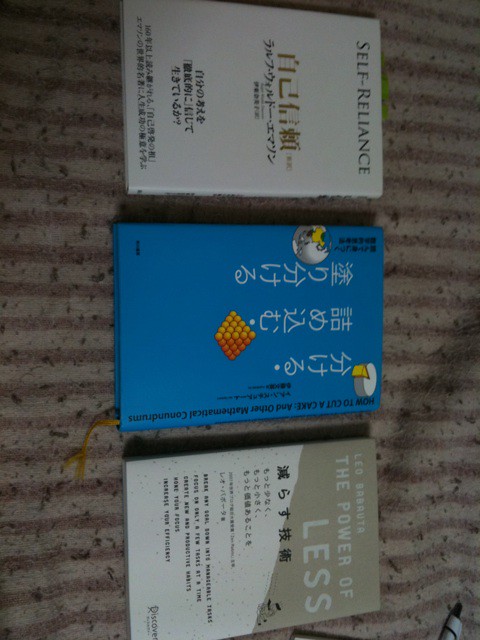The image showcases three horizontally arrayed hardback books against a background adorned with diagonal white and purple stripes. The topmost book is predominantly white, labeled "Self-Reliance" in English, alongside extensive Asian characters, likely Japanese or Chinese. The middle book is blue with an orange diagram resembling a pyramid made of circles, with additional Asian text. Notably, this book features a gold bookmark hanging out of it. The bottom book is half gray and half white, inscribed with "The Power of Less" in English at the top, followed by more Asian script. These books rest on a surface exhibiting brown and white tones, and a pen is observable at the bottom right of the image.